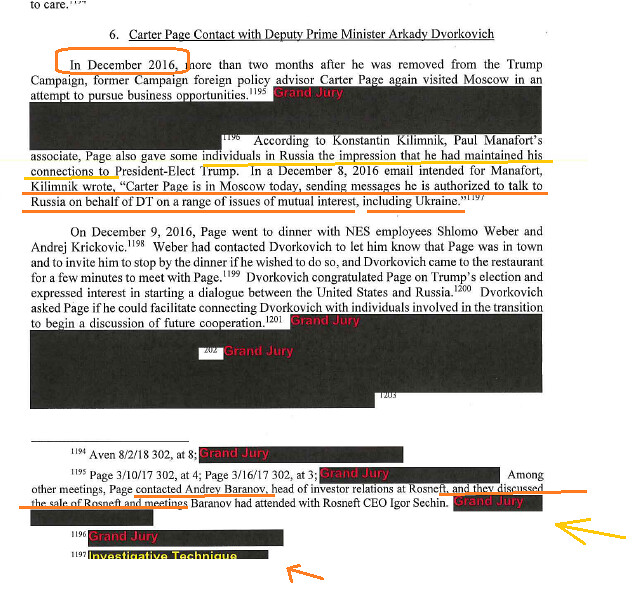This portrait-oriented image appears to be a heavily redacted court document or book page, primarily featuring black text on a white background, with several sections blacked out and labeled "Grand Jury" in red. An indented number six at the top marks a section titled "Carter Page Contact with Deputy Prime Minister Arkady Dvorkovich." There are multiple annotations in orange and yellow, including underlined sentences and arrows pointing to notable parts of the text. 

The visible text details that in December 2016, over two months after being removed from the Trump campaign, former campaign foreign policy advisor Carter Page visited Moscow to explore business opportunities. Konstantin Kilimnik, Paul Manafort's associate, reported in a December 8, 2016, email to Manafort that Page was in Moscow, claiming authorization to discuss a range of issues on behalf of President-elect Trump, including Ukraine. 

On December 9, 2016, Page dined with NES employees Shlomo Weber and Andrei Krikovich. Weber had informed Dvorkovich of Page's presence in Moscow, inviting him to join the dinner. Dvorkovich briefly attended, congratulated Page on Trump's election, and expressed interest in initiating U.S.-Russia dialogue. He also requested Page's assistance in connecting him with transition team members to discuss future cooperation. The document concludes with footnotes and additional redacted sections.